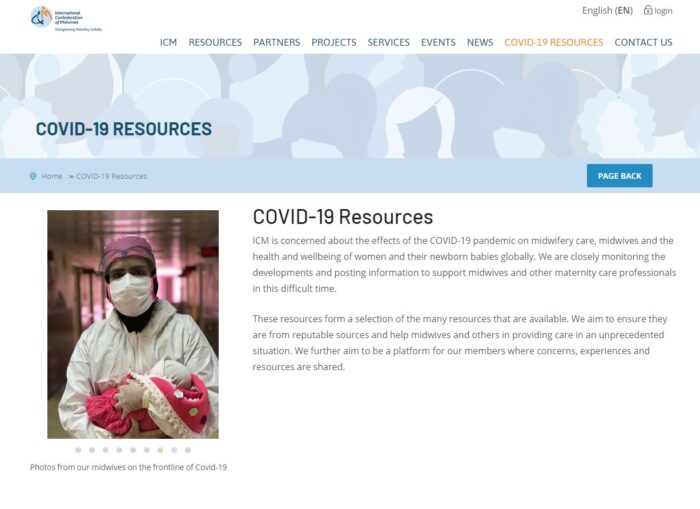This detailed caption provides a comprehensive description of ICM's COVID-19 webpage:

---

This is a screenshot of the International Confederation of Midwives (ICM) COVID-19 resource page. The top section features a white header bar separating it from the actual webpage. On the top left is ICM’s logo, which includes blurred text—likely stating "International"—in either blue or black. Next to this text is the ICM logo, depicting two simplified stick-figure-like individuals, one blue and one orange, standing side by side against a light blue background.

Moving towards the center-right of the header, there are navigation tabs labeled: 'ICM Resources', 'Partners', 'Projects', 'Services', 'Events', 'News', 'COVID-19 Resources' (highlighted in yellow), and 'Contact Us' (all other text in black). On the top right corner, there's an 'English' language option followed by a login icon.

Below the header, the main webpage begins. A blue banner stretches across the top, featuring drawn silhouettes of people in various shades of blue, gray, and white, depicting a background scene. Overlaid on this banner is the text "COVID-19 Resources" in bold blue.

Underneath this banner, there's a secondary blue divider. On the bottom left of this divider, text reads 'Home', followed by a right-pointing arrow and 'COVID-19 Resources'. On the far right side is a blue 'Page Back' button.

Further down the page, on the left side, there's an image of a person wearing a mask and a white lab coat or gown, holding an infant swaddled in a blanket. Below this image, the caption reads "Photos of our midwives from the frontline of COVID-19." To the right of the image, the text "COVID-19 Resources" serves as an introduction.

Continuing down, two black paragraphs provide additional information about ICM and their efforts, forming a detailed narrative on the organization’s involvement and resources provided during the COVID-19 pandemic.